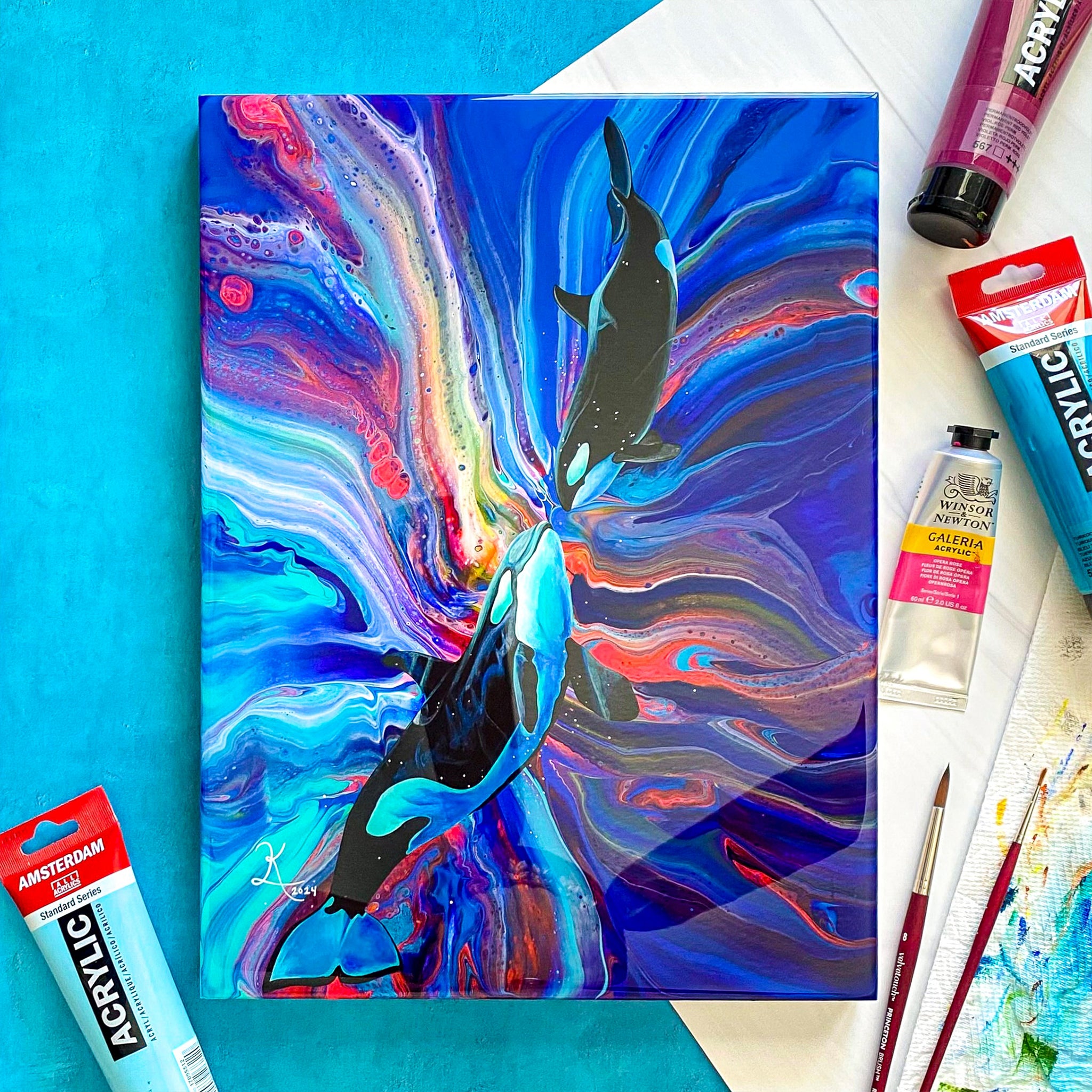In this vibrant and detailed painting, an artist beautifully captures a tender moment between two orcas, possibly a mother and her calf, as they swim nose-to-nose. The larger orca on the left looks affectionately at the smaller one on the right. Both whales are painted in striking black with hints of blue, seamlessly integrating with their modern, flowing forms. The background is an energetic swirl of colors, reminiscent of a more refined tie-dye pattern. It features a mesmerizing gradient that transitions from blues in the upper right corner to reds, purples, and oranges, eventually merging into neon hues of greens and whites on the left side. Surrounding the artwork are various artist tools, including tubes of Amsterdam and Winsor & Newton acrylic paints, and two well-used fine-tipped brushes. The entire composition exudes a sense of dynamic movement and emotional warmth, enhanced by the swirling backdrop and the expressive forms of the orcas.